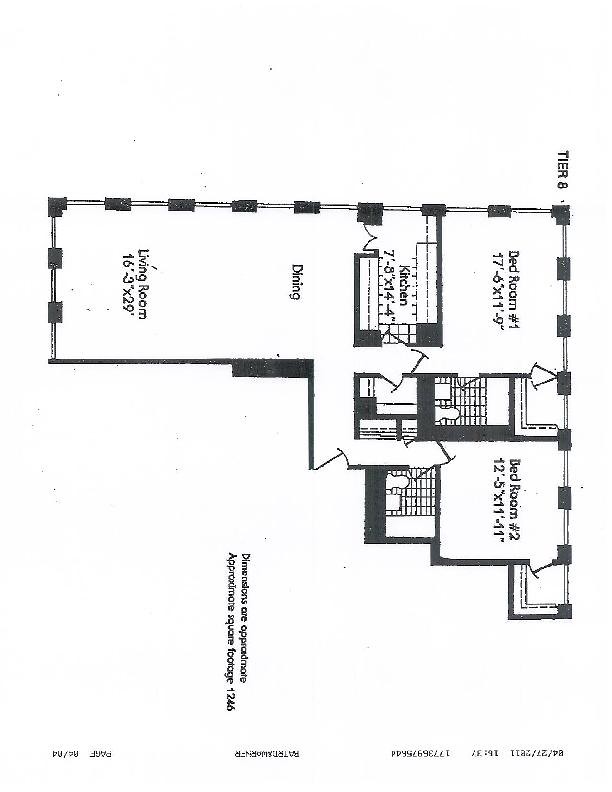This is an intricately detailed black and white blueprint of a home, oriented sideways requiring one to tilt their head to read the annotations. It is labeled "Tier 8." 

Upon closer inspection, the blueprint details a multi-room layout beginning with Bedroom 1 on the upper left. Bedroom 1 measures 17’ x 6’ x 11’ x 9’ and includes a closet. Adjacent to Bedroom 1, separated by a wall, lies the bathroom, and further alongside, you find Bedroom 2 measuring 12’ x 5’ x 11’ x 11’, also with an attached closet.

A hallway connects these initial rooms to the rest of the house. Proceeding down this hallway leads to an optional exit door, or alternatively, another hallway steering into the main section of the home. Turning left from this hallway, one enters the dining room, which extends further into the living room, sized 16’ x 3’ x 29’.

Heading right instead, the hallway branches into another small corridor, revealing entry points into a small closet and the kitchen. The kitchen, measuring 7’ x 3’ x 14’ x 4’, features a secondary access point leading into the dining room. Continuing further down this secondary hallway brings one to the main bedroom.

This blueprint provides a comprehensive overview of the home's layout, ensuring a clear understanding of room placements and measurements.